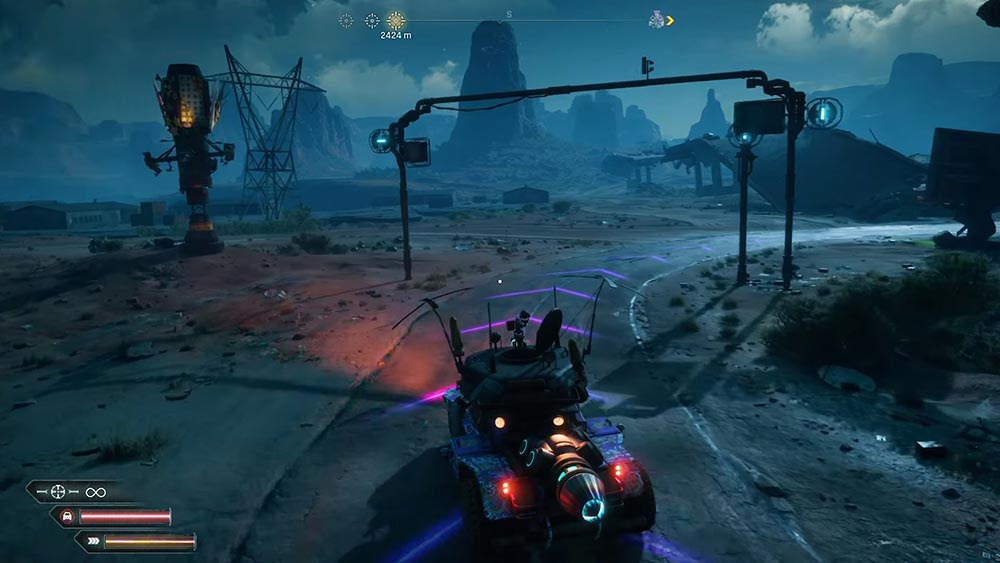The image is a highly detailed in-game screenshot from a video game, showcasing a post-apocalyptic landscape. The background features a gray, overcast sky with white puffy clouds and plateauing cliffs or large rock formations partially obscured by the moody atmosphere. The left side of the image displays a power line or electric tower alongside another black tower illuminated with lights. These structures rest on a dirt field scattered with some scrub and desert vegetation.

In the center of the image stands a black archway or overpass railing which frames a dirt road below. The road includes purple directional arrows pointing towards the right. Driving towards the foreground is a futuristic, rocket-powered truck with distinctive red taillights, purple lighting, and a silver cone at its center. The vehicle's design is sleek and modern, adding a vivid element to the somber environment. The overall setting is dark, gritty, and evocative of a desolate but intriguingly detailed desert climate.